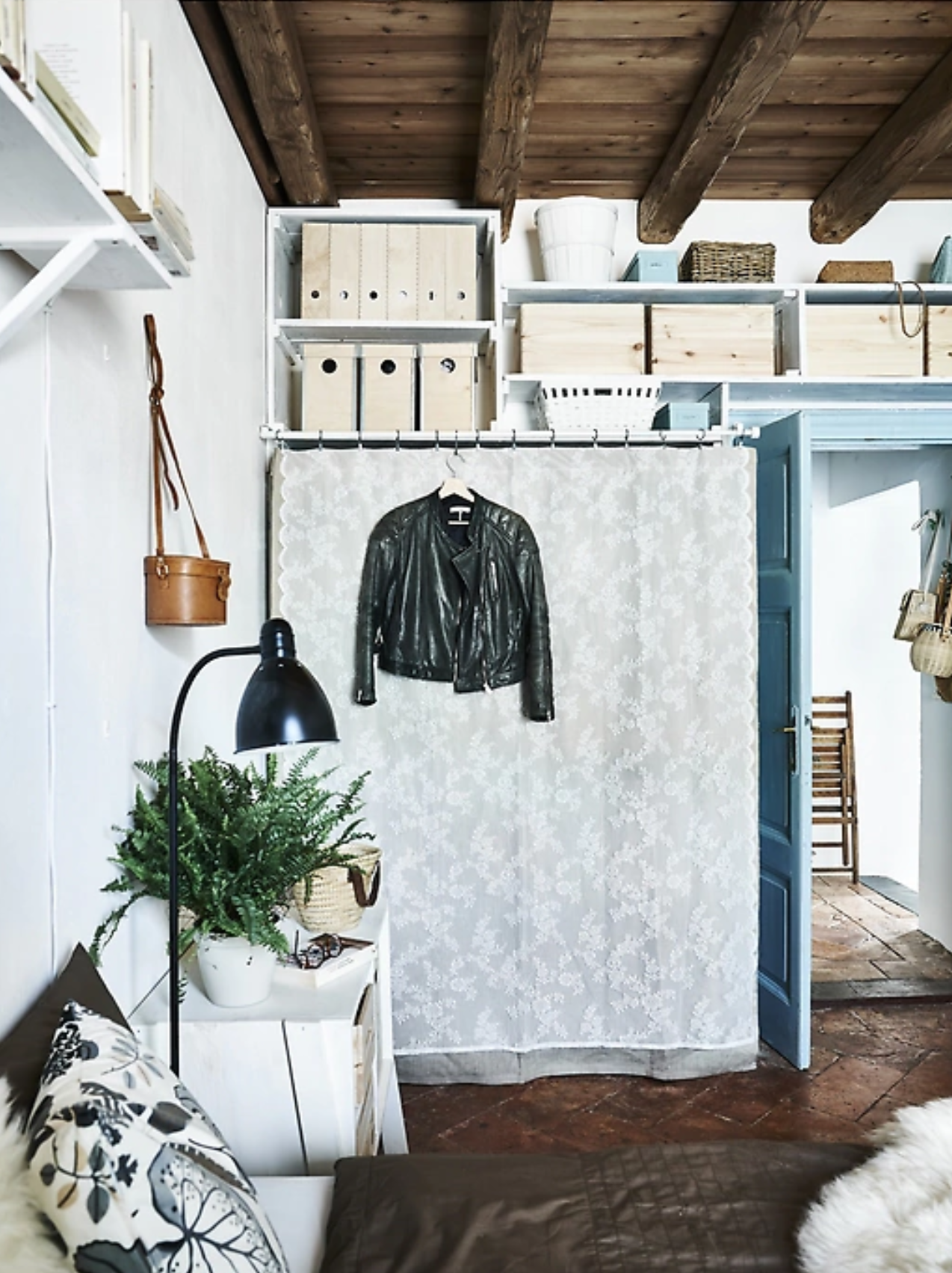The color photo captures a small room with a rustic charm, featuring a beam and plank wooden ceiling contrasted by white walls with blue trim. A visible blue door stands at the right rear, while a makeshift closet with either a drapery or shower curtain rod showcases a hanging black leather jacket on a wooden hanger. Above, shelves offer organized storage with wood-look boxes and basket organizers. To the left, a white wall houses a high bookshelf displaying various items, including a leather binoculars case hanging by its handle. Below, a piece of furniture—likely a couch or bench—shows a mix of throw cushions with botanical designs, a white sheepskin, and a brown cushion. Adjacent to this is a side table holding a potted fern, illuminated by a black floor lamp with a downward-pointing, old-fashioned street lamp-style shade. The room's floor appears to be brick or terracotta tile, and through an open doorway, light pours in from a window, revealing another room with chairs. The overall atmosphere is cozy and organized, with a detailed palette of blues, browns, blacks, whites, and greens enhancing its inviting feel.